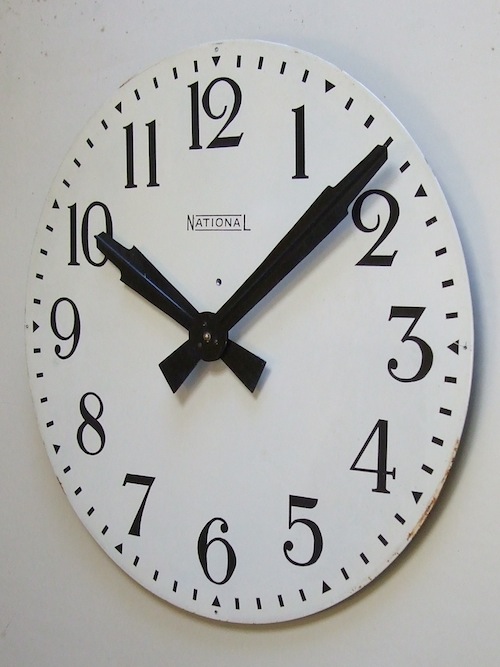The image features a close-up view of a circular wall clock set against a light gray backdrop. The clock's face is marked with bold black numerals, starting with 12 at the top and continuing sequentially around the clock's perimeter: 1, 2, and 3 on the right, 4, 5, and 6 at the bottom, 7, 8, and 9 on the left, and 10, 11, and 12 returning to the top. Each numeral is flanked by smaller dash markers at every 15-minute interval, denoting the time increments. The clock's short hour hand, also black, points to the 10, while the longer minute hand lies between the 1 and 2. Both hands intersect near the clock’s center, contrasting sharply against the light gray background.